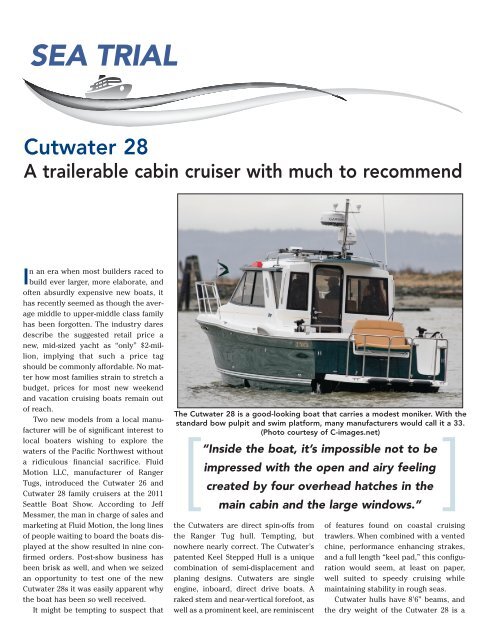The image is a page from a magazine featuring a section titled "Sea Trial," with an icon of a boat riding over waves. The main focus is a review of the Cutwater 28, described as a trailerable cabin cruiser with numerous commendable features. The centerpiece photo on the right side of the page shows a medium-sized motorboat named Cutwater 28, approximately 20-30 feet long, with a white enclosure and green hull, featuring an orange bench at the stern. The boat is equipped with an enclosed cabin, antenna on top, and glass windows, creating an open and airy atmosphere highlighted by four overhead hatches. Surrounding the photo is detailed text discussing the Cutwater 28’s unique design and appeal. The background includes a gray sky and trees, setting a serene scene for the boat. Below the photo, a caption reads: "Inside the boat, it's impossible not to be impressed with the open and airy feeling created by four overhead hatches in the main cabin and the large windows." Additional text emphasizes its practicality and affordability for middle to upper middle-class families, contrasting it with the expensive trends in the boating industry. The Cutwater 28’s innovative keel-step-hull combines semi-displacement and planning designs, offering stability in rough seas. It also highlights the success and high demand observed at the 2011 Seattle Boat Show, with Fluid Motion LLC securing nine confirmed orders.